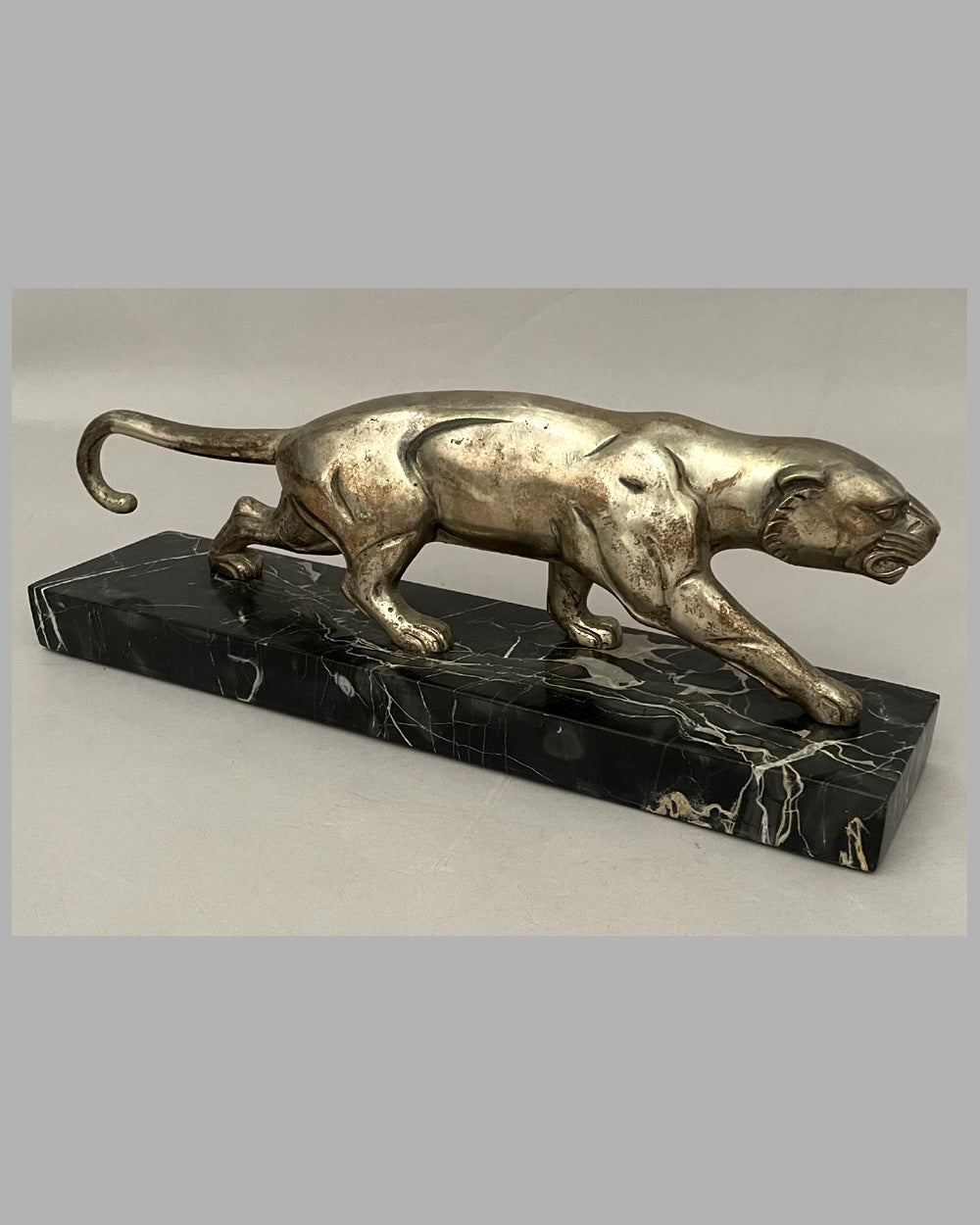The image portrays a detailed, realistic photograph of a decorative statue, which appears to be a beautiful gold jaguar or panther figurine. The luxurious, gold-colored jaguar is intricately detailed, possibly hand-carved, and measures approximately 8-10 inches in length. The figurine is depicted mid-stride, with all four legs, its tail, and its face meticulously crafted to embody a lifelike appearance. This elegant sculpture is mounted on a rectangular, black marble or granite platform featuring striking gold or white marbling throughout its surface, enhancing its sophisticated aesthetic. The platform and statue together create a refined piece that would make an exquisite desk ornament or paperweight. The background of the overall image is gray, while the image within the image showcases the statue against a beige stone-like backdrop, suggesting that this might be a photograph of a printed picture.